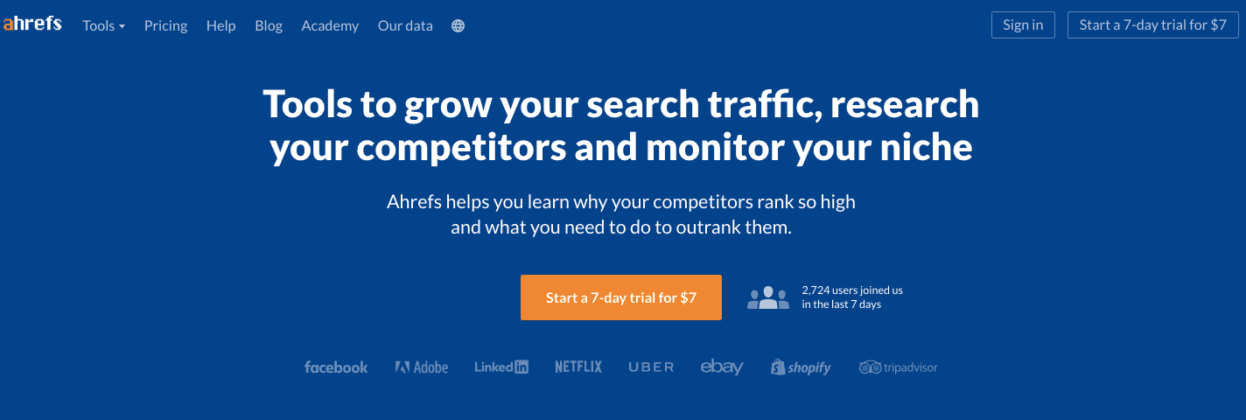The image appears to be a screenshot of the Ahrefs website. The header features the Ahrefs logo, with the 'A' in orange and the remaining letters in white. Adjacent to the logo, there are several clickable options: "Tools" which has a drop-down menu, followed by "Pricing," "Help," "Blog," "Academy," and "Data," each without a drop-down menu. There's also a globe icon indicating language or region settings.

On the right side of the header, there are options to "Sign in" or "Start a 7-day trial for $7."

The main body of the webpage has a bold headline that reads, "Tools to grow your search traffic, research your competitors, and monitor your niche." It further explains, "Ahrefs helps you learn why your competitors rank so high and what you need to do to outrank them."

Below this, there is a prominent orange button that says, "Start a 7-day trial for $7." Accompanying this button is a small illustration depicting three people. Nearby, there is text stating, "2,724 users joined us in the last 7 days."

At the bottom of the image, logos of prominent companies are displayed, including Facebook, Adobe, LinkedIn, Netflix, Uber, eBay, Shopify, and one more that is not legible.